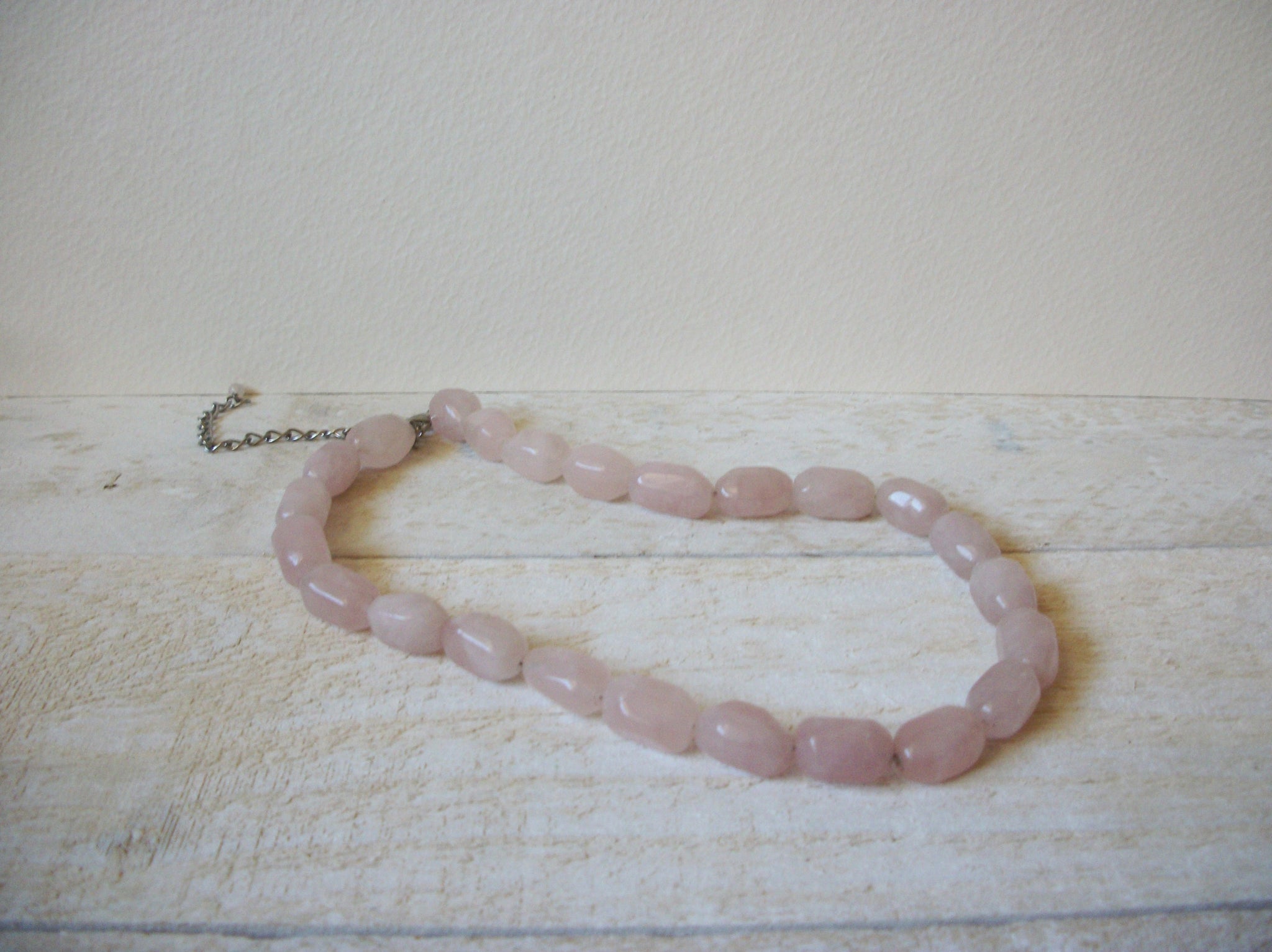This is a detailed photographic image of a beaded bracelet lying on an off-white, lightly marked wooden surface. The bracelet is composed of light pink, cylindrical beads that resemble pink pearls. There is a small silver chain extending from one end of the bracelet, partially visible in the image. The beads are uniformly sized and arranged in a loop. In the background, a plain white wall with a slightly textured surface can be seen. The composition of the image emphasizes the delicate contrast between the soft pink hues of the bracelet and the neutral, earthy tones of the wooden surface. No text is present in the image.